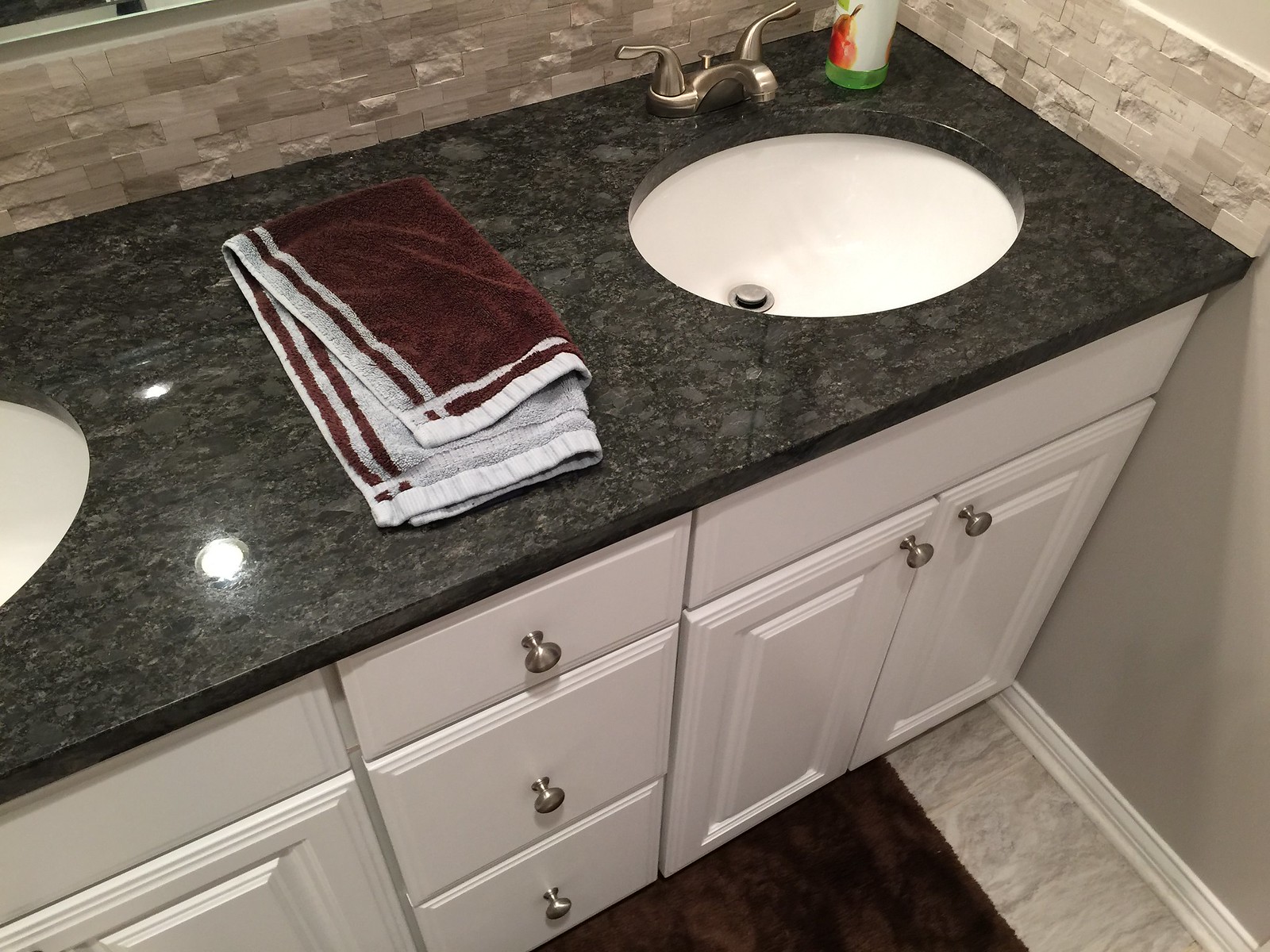The image captures a detailed view of a bathroom counter from above. On the left, half of a circular white sink is visible, paired with a sleek black countertop. The countertop features two bright white circles of light reflecting off its surface. Central to the composition is a neatly folded burgundy and gray striped towel. The sink itself is deep and white, complemented by a silver faucet positioned at the top.

The backsplash area behind the sink consists of a mosaic of brown and darker brown square tiles, adding a touch of warmth and texture to the setting. A spray bottle, partially visible, stands on the counter, adorned with an image of fruit at its base.

Moving downward, white cabinets with three stacked drawers come into view, each equipped with small circular silver knobs, contributing to the bathroom’s clean and modern aesthetic. At the bottom of the image, a dark brown bathroom rug contrasts nicely against the adjacent gray floor. The bottom right of the photo also reveals a portion of a gray wall, completing the balanced and organized look of the bathroom.